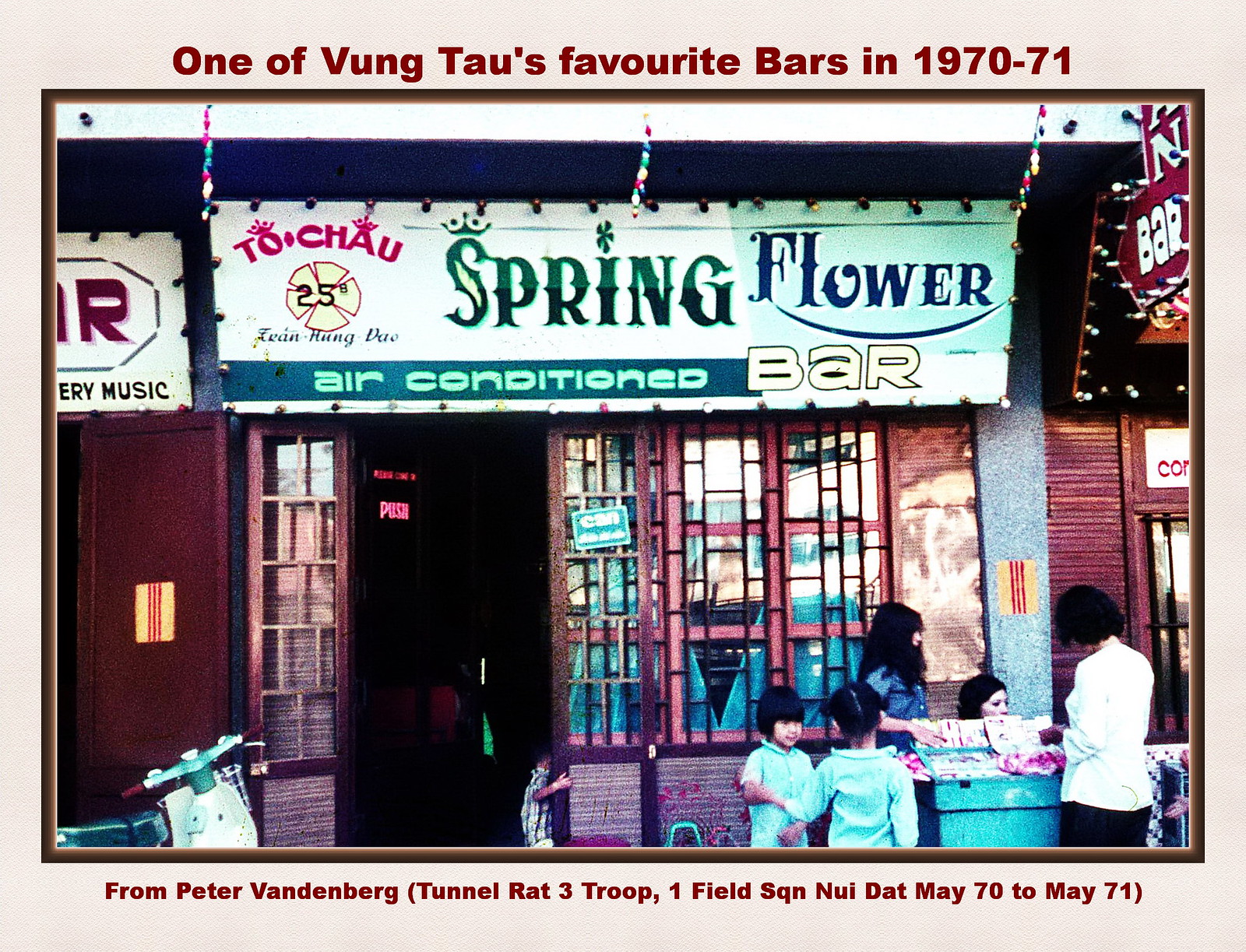In this detailed photograph set against a white-pink background with a brown border and a tan frame, we see a bustling street scene in Vietnam, specifically Vung Tau. The image is fronted by a little shop with a prominent sign above it reading "To Chau Spring Flower Bar," noted as being air-conditioned. The storefront features vertical windows with small square insets, adding an older architectural feel. In front, a small stand or display attracts attention, with a woman dressed in a short white blouse over black pants engaged in bartering or conversation. She is accompanied by two children wearing blue jerseys, standing close by. Behind the display stand, another woman dressed in a blue top with long dark hair interacts with a seated woman, who also has dark hair. In the lower-left corner of the photograph, a blue and white motorbike is parked, suggesting a lively, everyday street ambiance. Overlaying the photo, red text frames a historical note: "One of Vung Tau's favorite bars in 1970-71," with attribution below: "From Peter Vandenberg (Tunnel Rat 3 Troop, 1 Field SQN, Nui Dat, May 70-May 71)." The sign and descriptive elements highlight the image's likely significance and nostalgic value.